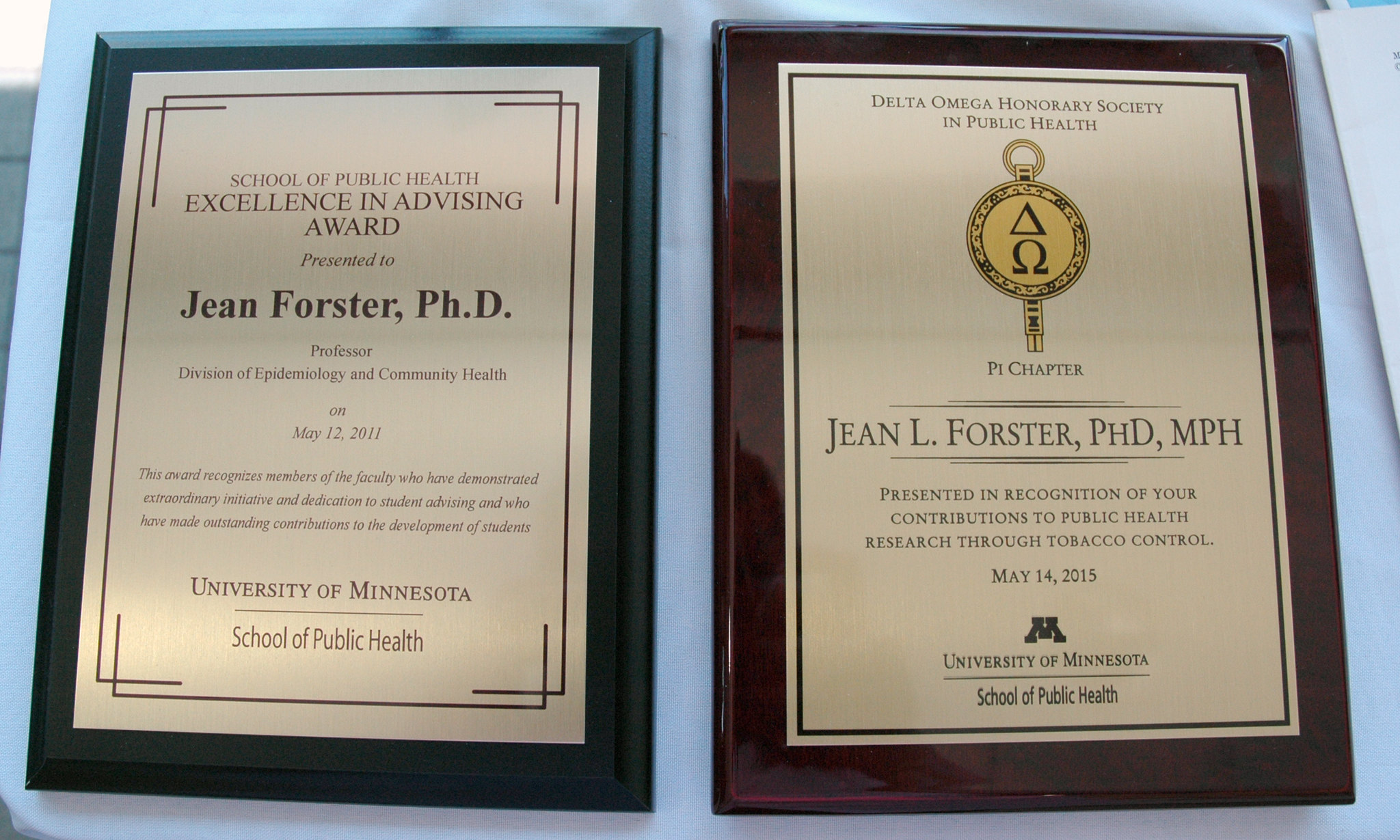This image shows two plaques mounted on a wall, each framed in dark brown. Both plaques honor Gene Forster, Ph.D., for his contributions to the field of public health. The plaque on the left, titled "Excellence in Advising Award," was presented by the University of Minnesota School of Public Health to Gene Forster, Ph.D., on May 12, 2011. The plaque features an off-white background with bold brown text and recognizes his outstanding advising. The plaque on the right, titled "Delta Omega Honorary Society in Public Health," acknowledges Gene L. Forster, Ph.D., M.P.H., for his significant contributions to public health research through tobacco control. This award, presented on May 14, 2015, by the same university, also features an off-white background with brown text and includes the Delta Omega Honorary Society logo. Both plaques emphasize his significant impact within the School of Public Health at the University of Minnesota.